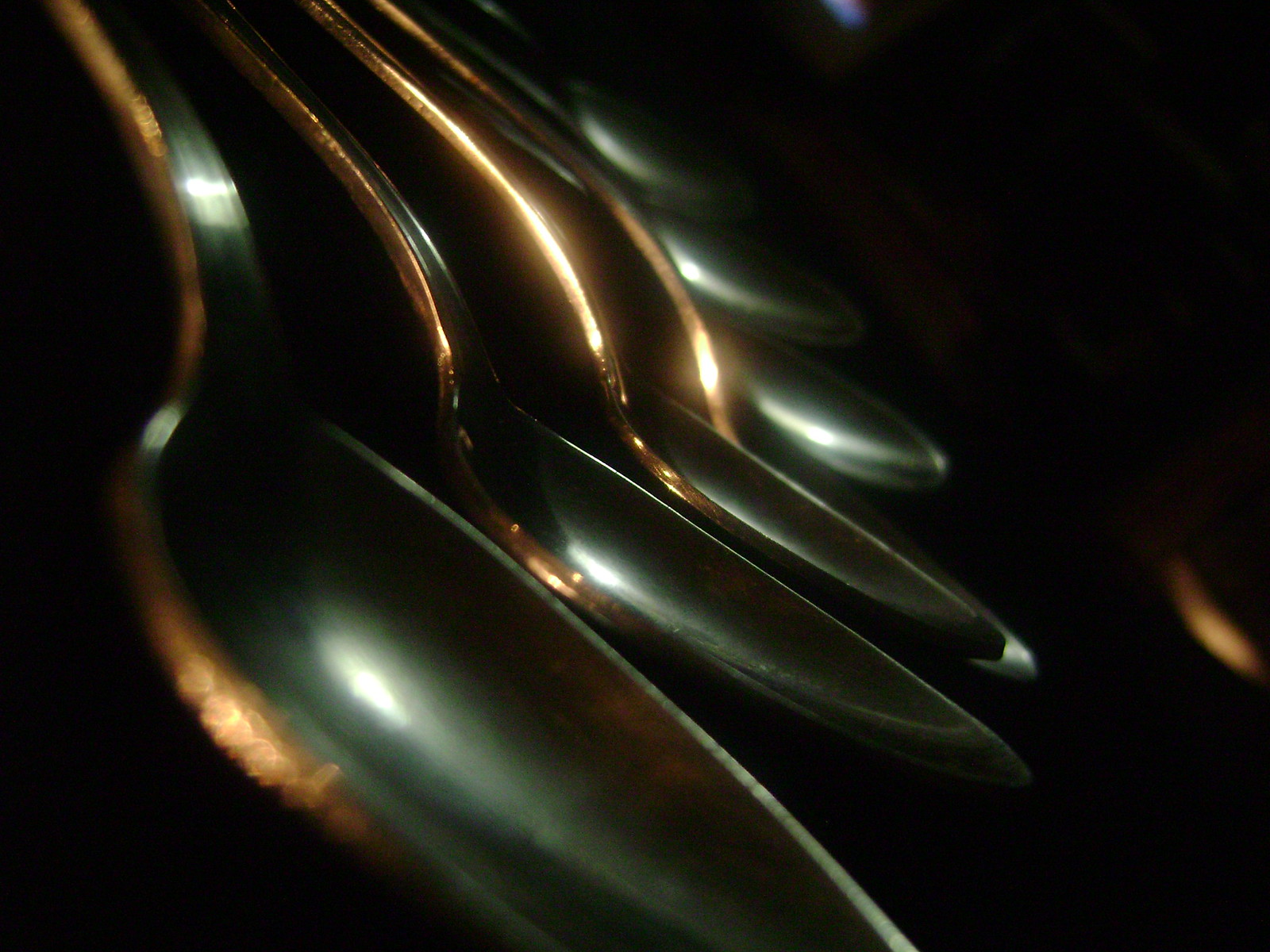This close-up, highly focused photograph captures an artistic arrangement of seven steel spoons on a dark, featureless black background. The spoons, which appear to have an antique gold plating, create a soft, brassy hue under the light, adding a rich warmth to their shiny, steel-like surface. The spoons are arrayed in a slightly curved, spiraling pattern, with their oval-shaped bowls and part of their handles visible, all pointing towards the right. The image composition leads from an oversized, highly detailed foreground spoon to increasingly blurry and smaller spoons receding into the distance, enhancing the sense of depth. The photo's lighting, seemingly sourced from below and to the right, casts reflective highlights across the deepest parts of the spoons' bowls, further emphasizing their curvature and sleek design. There's a subtle blue reflection at the top, contributing to the overall monochromatic and minimalist aesthetic of this visually intriguing still life.